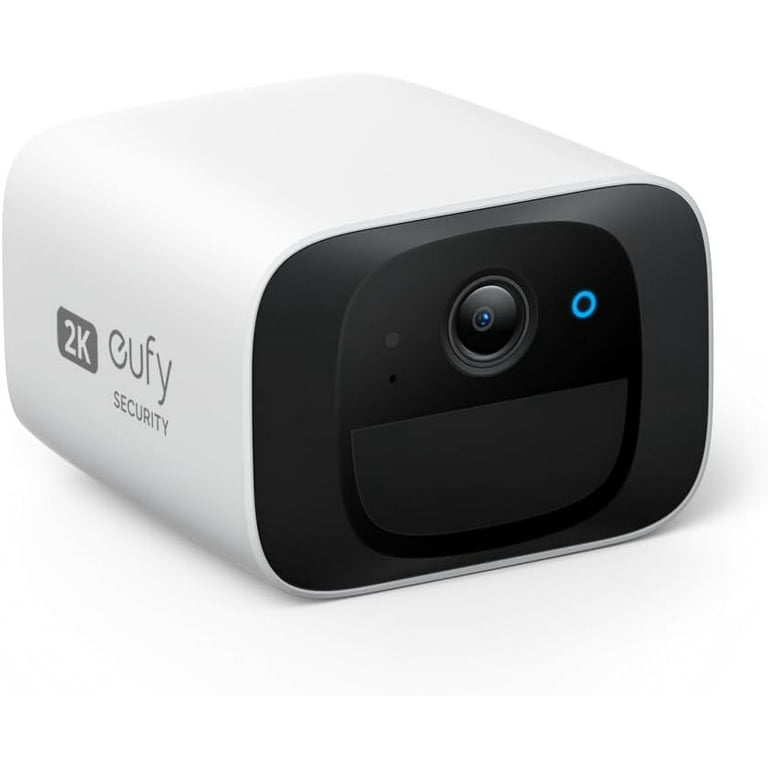The image displays a security camera from the brand Eufy, specifically marked with "2K" Eufy security. The device is shaped like a rectangular cubic box with rounded edges and sides. The housing of the camera is white, while the front panel, which faces the viewer, is black. At the center of this black panel, there's a prominent camera lens. To the right of the lens is a small blue LED indicator, and to the left is another small hole, possibly for an infrared emitter or focusing technology. Beneath these components, there is a U-shaped, matte black section. The camera is tilted slightly to the right, casting a shadow, and is set against a white background.